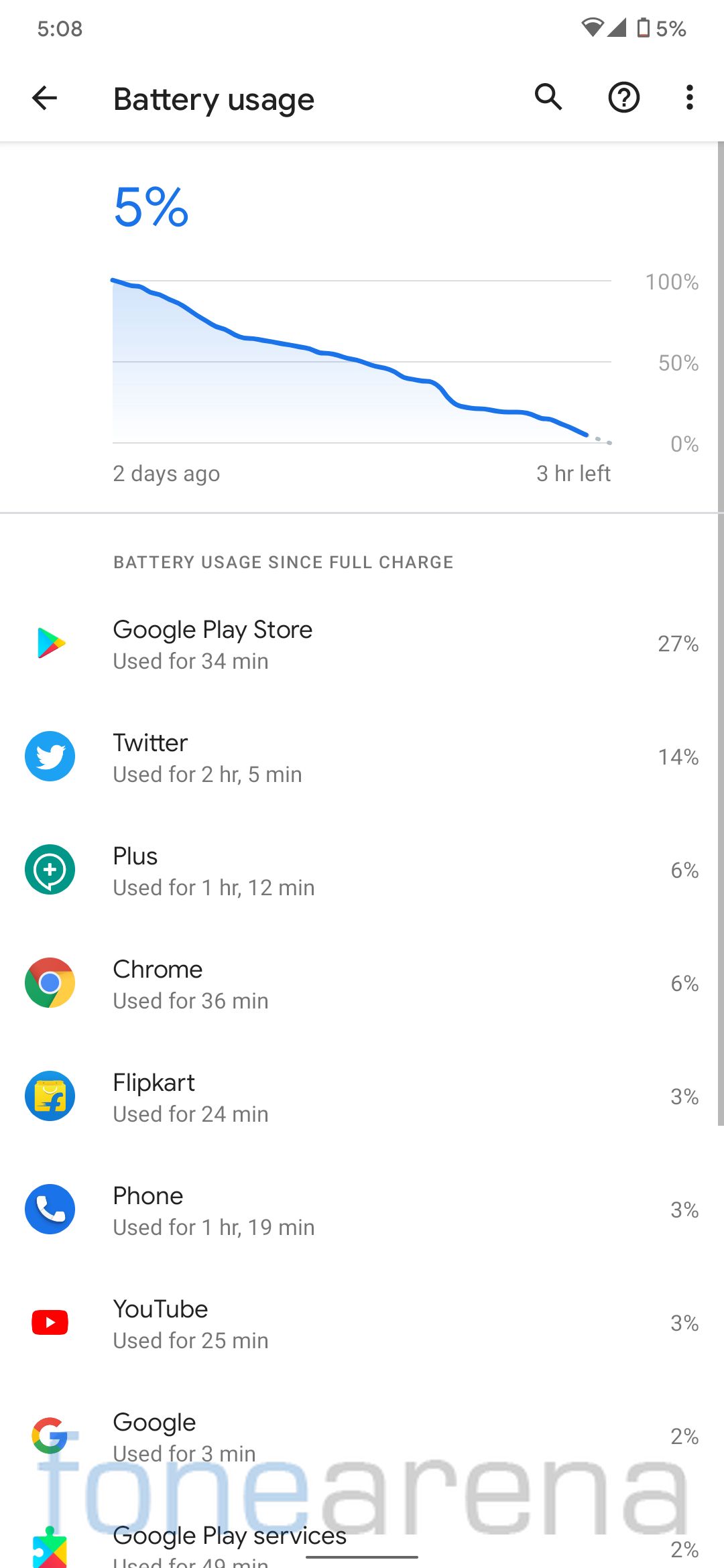This screenshot displays an Android phone's battery usage statistics. Captured at 5:08 PM with the battery at 5%, the image shows the "Battery usage" section, complete with a search bar, a question mark icon, and a three-dot menu for additional options. Directly below, the screen indicates the current battery level of 5% and features a detailed graph charting the battery depletion from 100% over the past two days. The graph estimates that the device has about three hours of battery life remaining.

Further down, the usage statistics since the last full charge are listed, showing:
- Google Play Store: 34 minutes (27%)
- Twitter: 2 hours 5 minutes (14%)
- Plus: 1 hour 12 minutes (6%)
- Chrome: 36 minutes (6%)
- Flipkart: 24 minutes (3%)
- Phone: 1 hour 19 minutes (3%)
- YouTube: 25 minutes (3%)
- Google: 3 minutes (2%)
- Google Play Services: 49 minutes (2%)

Overlaying the screenshot is a watermark that reads "PhoneArena."